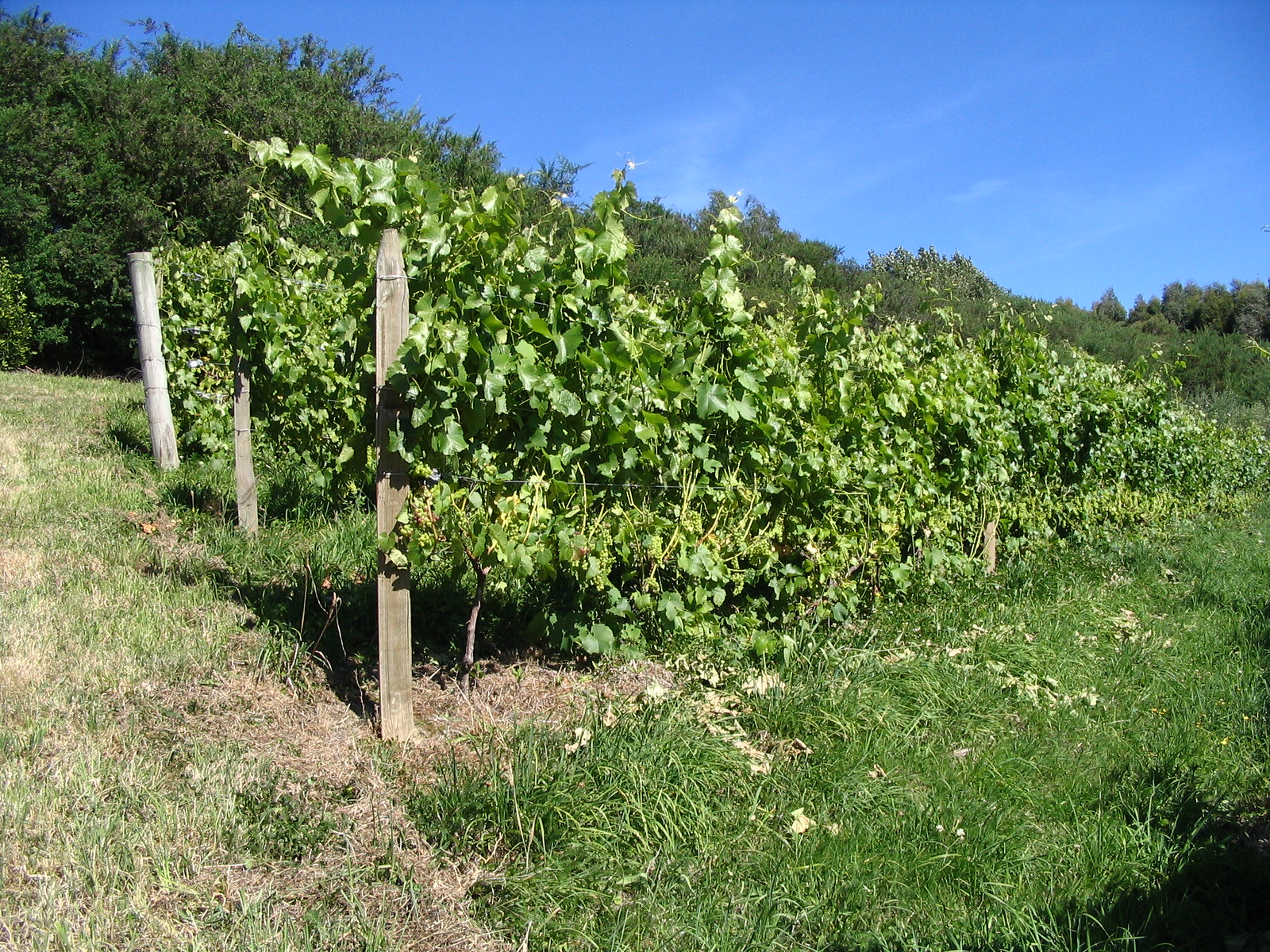The photograph captures a vibrant outdoor scene on a very bright, sunny day with a vivid blue sky and a few wispy, cirrus clouds scattered throughout. At the top, tall green trees with lush leaves create a backdrop that almost touches the upper edge of the image. Moving down, three wooden posts align horizontally, rising from what appears to be a grassy hillside. Emerging from these posts are tall, leafy green plants, potentially part of a small vineyard, though it's not evident what specific plants are growing. The ground around these plants is a mix of verdant green grass and patches of drier, lighter brown grass, particularly on the left side. This idyllic setting combines the vibrant growth of the vines with the lush, natural backdrop of trees and a beautifully clear sky.